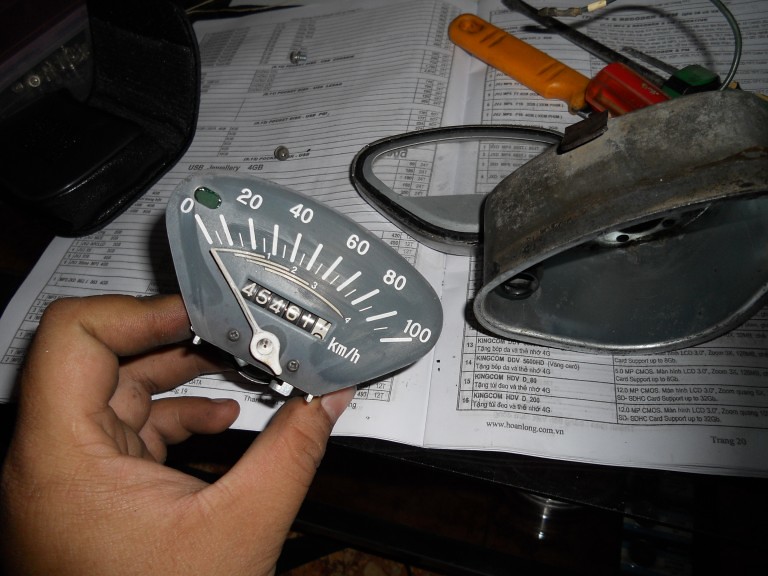A man is depicted in a dimly lit setting, meticulously holding up a disassembled speedometer, likely from a motorbike. In front of him lies a bilingual manual, possibly in Vietnamese and English, as indicated by a visible .vn domain hinting at Vietnam. The manual is open to a page filled with specifications and numbers, serving as a reference guide. Strewn across the surface are various tools, including a screwdriver and a small hacksaw, suggesting the intricate process he undertook to dismantle the speedometer. The housing and glass cover of the speedometer have been carefully removed, revealing that the odometer reads 45,401 kilometers. The scene captures a moment of detailed mechanical engagement, highlighting the man's skill and precision in working with motorbike components.